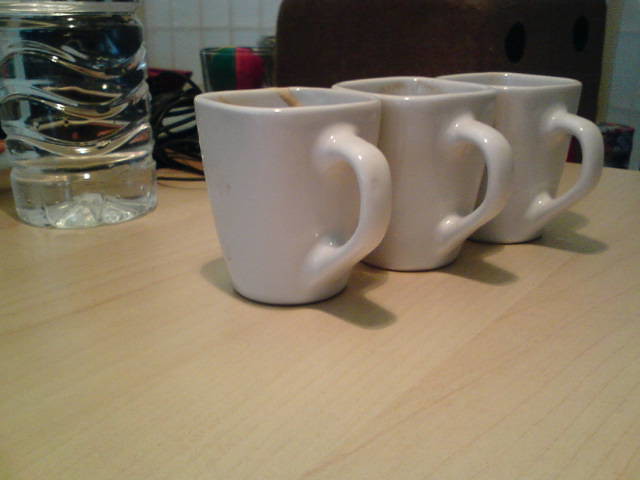The photograph showcases a blonde wood countertop featuring three identical ivory off-white ceramic mugs as the focal point. These heavy mugs are square on top with rounded edges and aligned closely together, side-by-side with their handles facing the camera, casting grey shadows on the countertop. The mugs appear to be stained brown or tan inside, suggesting they previously held coffee. In the background to the left, there's a clear plastic bottle of water with about an inch of water remaining, characterized by decorative swirls. Beyond that, the image reveals a white tile wall partially obscured by various dark objects, including some computer cables and a cup filled with neon-colored pink and green items of unclear nature. Further to the right, a red and green bowl and a dark brown chair with armrests add additional background detail.